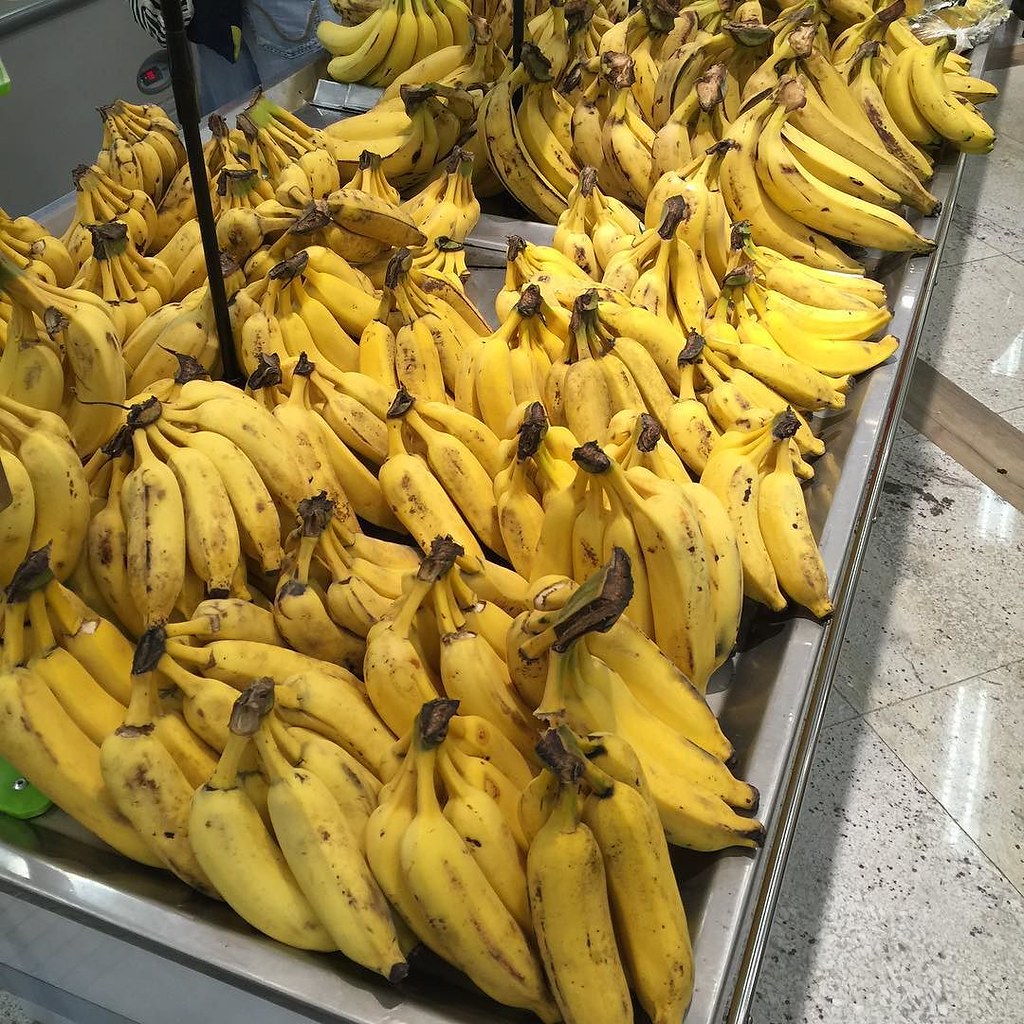This photograph is taken inside a grocery store and prominently features a large display of bananas. The linoleum floor tiles are visible, marked by a cord covered for safety. The polished, dotted floor is typical of supermarket aisles. The bananas, arranged in bunches of three to five, stretch diagonally from the lower left to the upper right corner, dominating the majority of the frame. They are long, uniform, and appear genetically modified, but many are bruised and overly ripe. A large, gray metal tray holds the bananas, though it's barely visible under the sheer quantity of fruit. Amongst the bananas, a single black rod is noticeable, though obscured by the abundance of produce. In the background, the lower half of a person’s pants can be seen, cut off from the rest of the picture. The floor around the display seems slightly dirty, adding to the everyday realism of the scene.